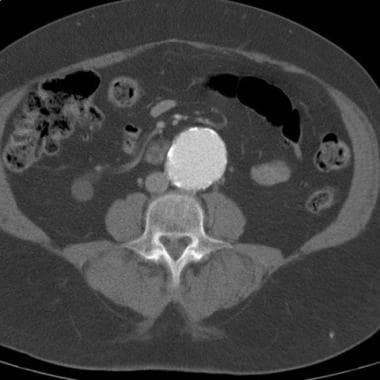This grayscale MRI scan of a brain features intricate structural details. Dominating the image is a centrally highlighted circular region, surrounded by various shades of gray. Just above the central highlight is a distinct white circle, likely indicative of a significant anatomical feature. The image also reveals two prominent voids or black regions in the top left and right corners, with additional smaller black and dark gray splotches scattered throughout. The bottom part of the scan appears gray, with a possible outline that may include the brain stem. The intricate swirls and miscellaneous structures, all framed by a black background, are void of any labels or annotations, emphasizing the raw medical data captured in this sectional MRI.